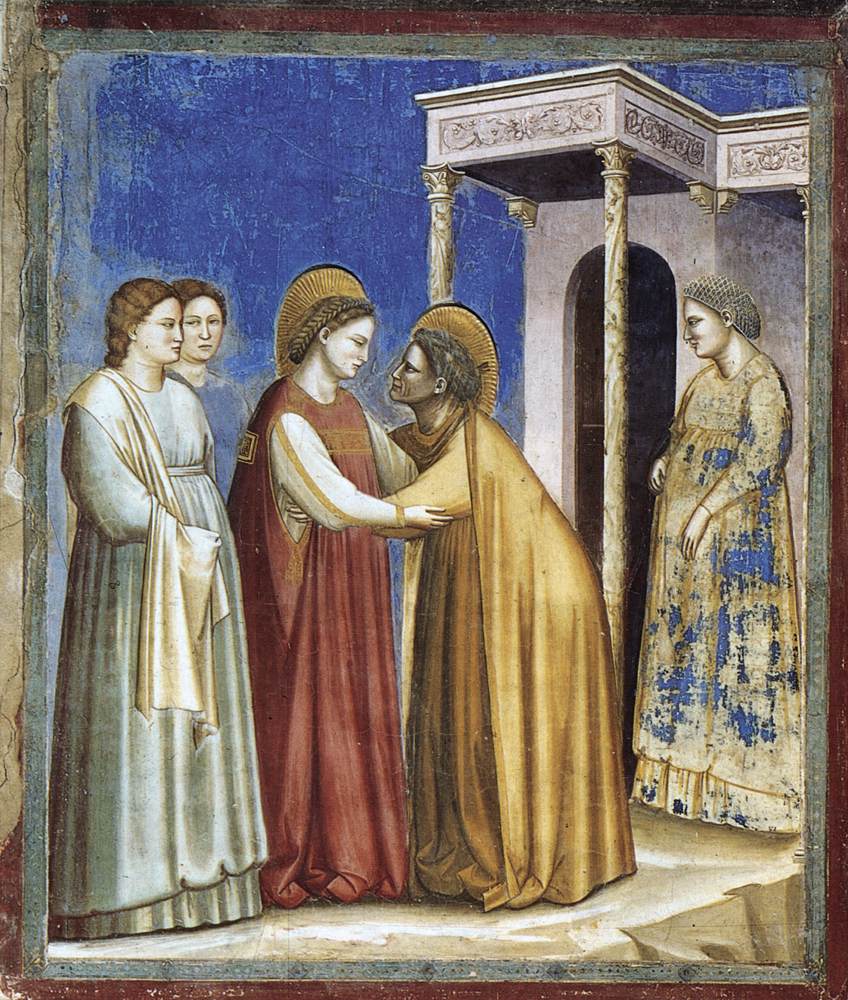The image depicts a Renaissance-era fresco painting, attributed to artist Giotto di Bondone, titled "Number 16, Scenes from the Life of the Virgin, Number 7, Visitation" from 1306. The painting features five people set against a blue sky, bordered by a building with an archway and columns. The architectural structure behind them includes ornamental carvings and artwork, with a curved top edge above the door. In the center, the Virgin Mary and Elizabeth, both in long garments, are embracing each other with serious expressions as they stare into each other's eyes. On the left, two women in bluish-gray robes with hair pieces are observing the scene without visible facial expressions. On the right, a woman in a blue and white dress stands with a serious look, her body turned slightly to the side, gazing straight ahead. The entire scene is framed by a dark black-brown border, followed by a bluish-grayish inner border.